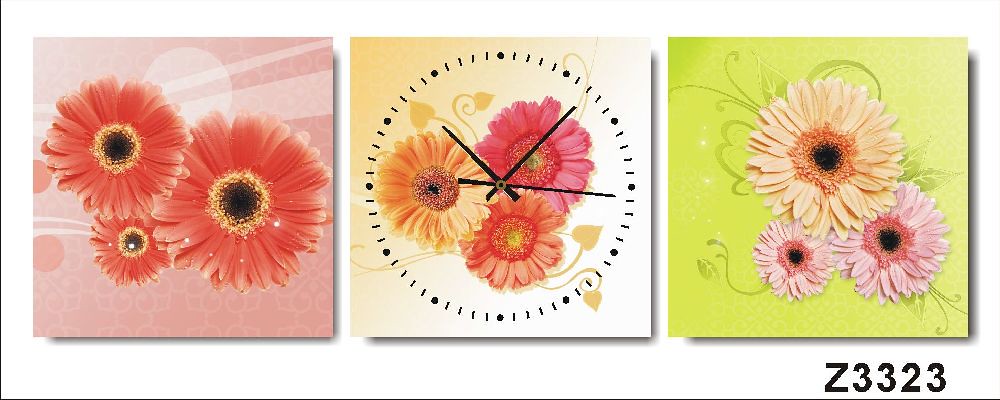The product image displays three square paintings or prints arranged in a row, each showcasing a floral design with three bloomed flowers viewed from above, revealing their brown centers. The left painting features a pinkish background adorned with pink flowers and subtle circles and lines. The central piece, a functional clock with a yellow background, depicts one pink and the other two flowers in orange and yellow; it features black hands marking approximately seven minutes after ten, with dots and lines indicating time in place of numbers. The rightmost painting presents a light green background, highlighted by decorative vines and swirls. This image shows similar flower designs, with a prominent yellow flower at the top, and two pink flowers at the bottom. Both a thin horizontal line along the bottom and a vertical line on the left side frame the composition. The code "Z3323" is also visible in black in the lower right corner of the rightmost painting.